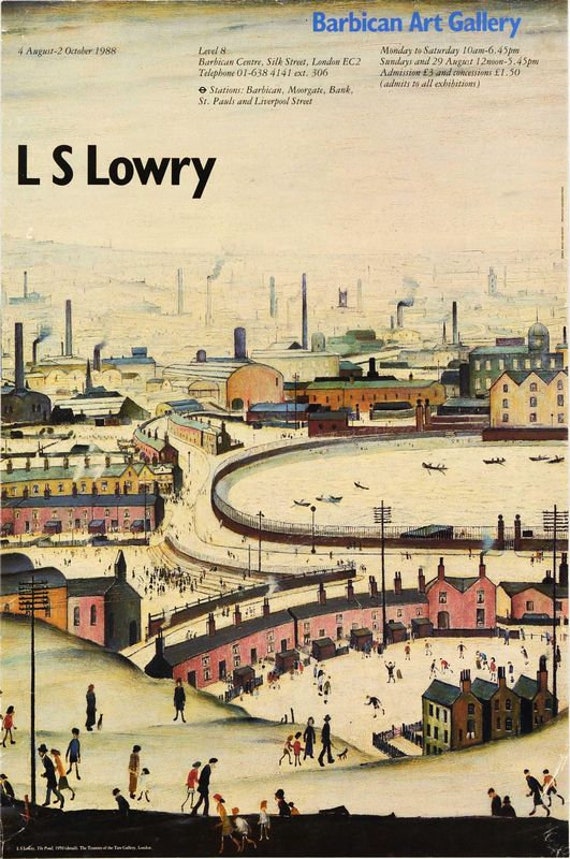A detailed poster in an older-style, up-close photograph depicts information about an exhibition at the Barbican Art Gallery. In the topmost section, 'Barbican Art Gallery' is prominently displayed in blue text, detailed with smaller, italicized black text that outlines the gallery's address: Level 8, Barbican Centre, Silk Street, London, EC2, and includes additional information likely regarding opening times and contact details. In the upper left corner, the dates "August 2 to October 1988" are evident, showcasing the limited run of the exhibit.

Beneath these details, in larger black text, the artist's name L.S. Lowry is highlighted, indicating that the artwork featured is by this renowned artist. The image on the poster itself is an intricate, aerial view of a town bustling with activity. The landscape includes a mix of residential rooftops and industrial elements, such as tall smokestacks emitting smoke. A lake with gondola-type boats cuts through the middle, adding a serene touch amidst the busy town scene. The foreground is vibrant with tiny human figures walking and interacting. This townscape illustration, seemingly part of a larger work by L.S. Lowry, effectively captures the essence of urban life and industrial vigor.